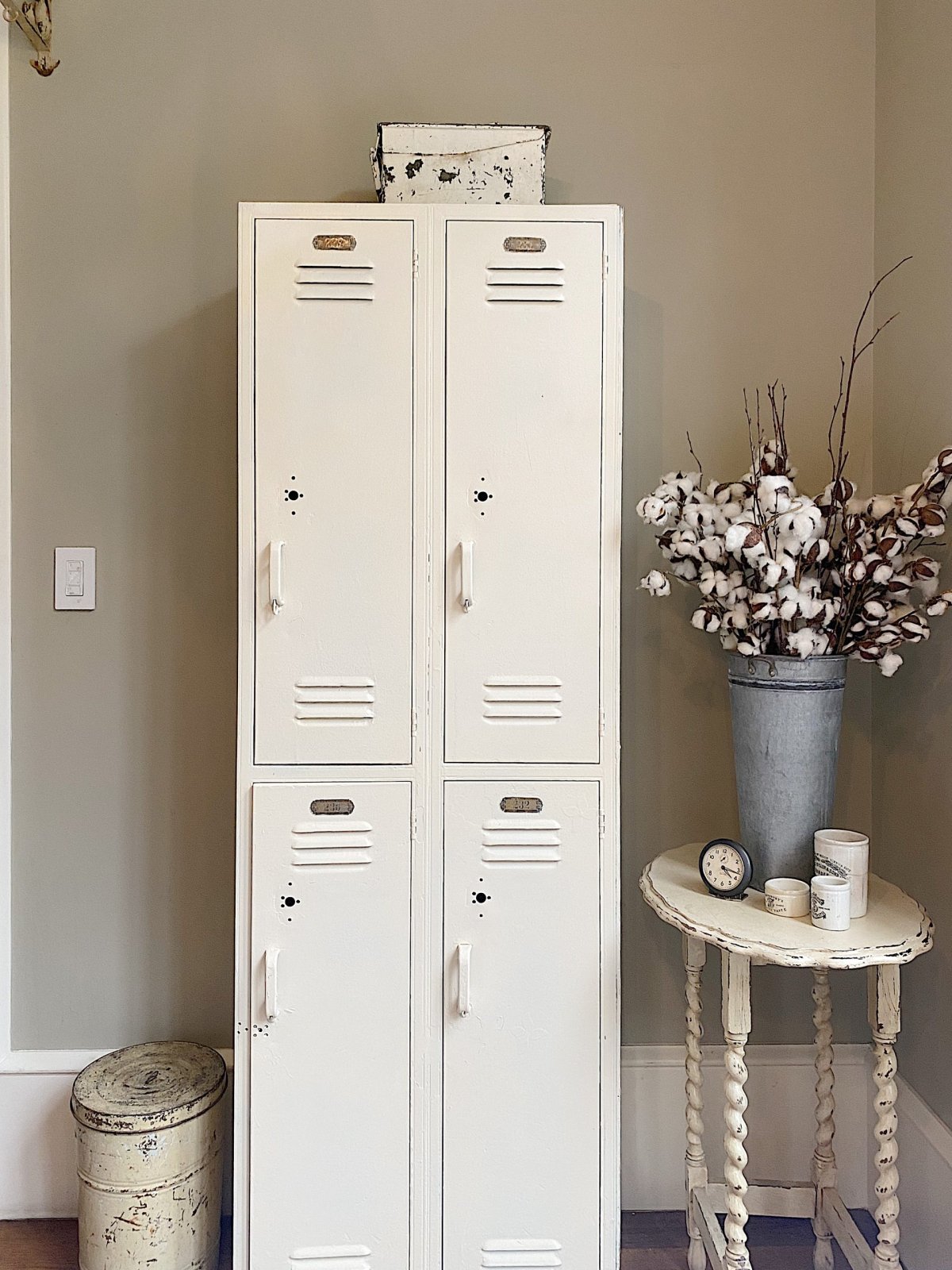The image depicts a room with a detailed setup. The back wall, extending down about four-fifths of the page, has a white, grayish-brownish color. There is a white push-kind light switch halfway down the picture on the left side, slightly off the left edge of the page. Along the bottom of the wall, a thick white border runs all around, and just above the bottom edge, some brown flooring is visible.

On the left side, in front of the border, there is a beat-up and rusty white trash can with a white lid. Moving to the right, there are four white lockers in a two-by-two arrangement—two on top and two on the bottom—extending almost to the top of the page. Each locker features a silver plate at the top and ventilation slits, with three black slits above and below the plate. Atop the lockers, there is a small, white box with black splotches, resembling an army ammunition box.

To the right of the lockers, nearly off the right side of the page, sits a white oval-shaped end table with four spiral legs and a flat, somewhat beat-up white top marked with black spots. On this table, a tall, skinny, silver aluminum vase contains white and black flowers, possibly resembling cotton plants with cotton bolls. In front of the vase and to the left sits a small alarm clock. Alongside the alarm clock are two small ceramic crocks, each with black markings on the front. The crock farthest to the right is slightly bigger. Behind the smaller crocks and to the right of the vase is a third, larger white crock with black markings, roughly twice the size of the others.